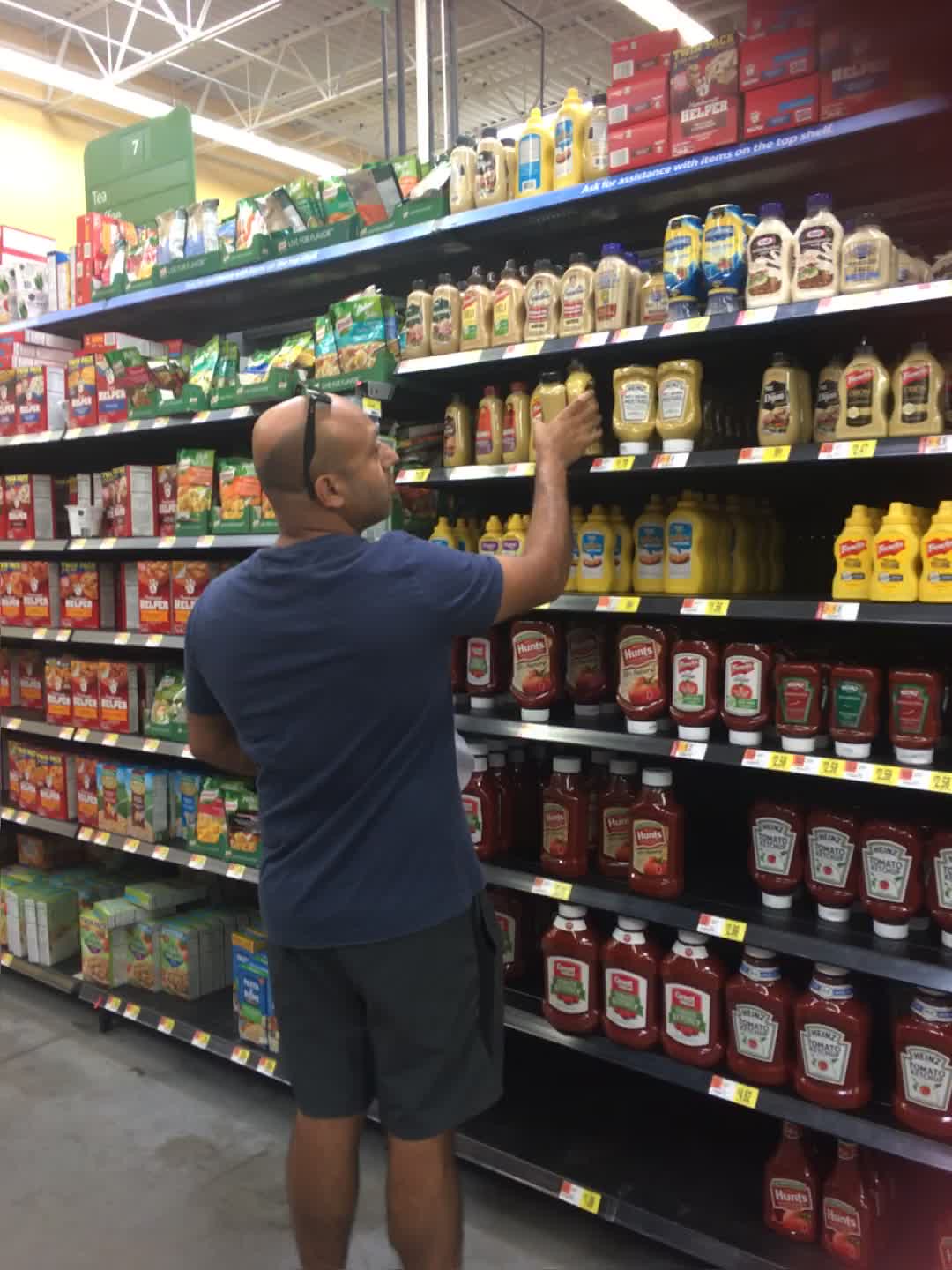This rectangular image, oriented with the longer side running vertically, captures a scene inside a grocery store, specifically in the condiment section. The photograph features a man of ambiguous ethnicity with a slight brown complexion, wearing a dark blue t-shirt and gray shorts. He is bald, and a pair of black sunglasses, resembling Ray-Ban Wayfarers, rest on top of his head. The man is reaching upwards to grab a bottle of golden-brown mustard from one of the higher shelves. His stance reveals a profile view as he looks over his right shoulder at the various products. Below the mustard he's reaching for, the shelves display an assortment of other mustards, with common yellow mustard in bright plastic bottles. To the upper right, some mayonnaise jars are visible, and ketchup bottles fill the lower shelves, some of which are designed to stand on their caps for easy dispensing. An empty shelf can be seen at the very bottom. The shelves in front of him are part of a tall, multi-tiered unit, approximately eight feet high, housing various condiments and other items. The left side of the aisle contains more grocery products, though they are not clearly identifiable. The store's flooring is gray concrete, complemented by white latticework on the ceiling and yellow-painted walls, with fluorescent lights illuminating the scene from above.